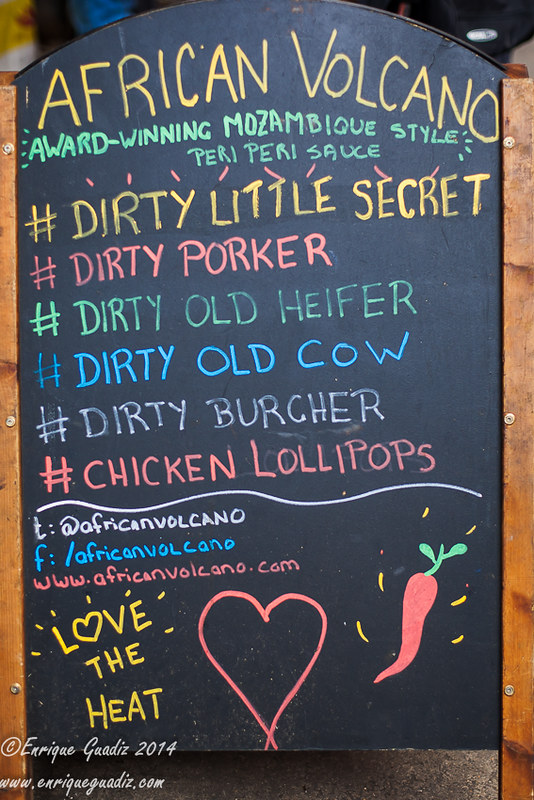This color photograph, taken in portrait orientation, features a black chalkboard menu, framed with arched wooden sides, commonly seen in front of cafes. Handwritten in vibrant colored chalks—yellow, green, blue, pink, and orange—the chalkboard prominently displays "African Volcano" at the top, followed by the smaller, detailed phrase "award-winning Mozambique style peri-peri sauce." Below this, there are six colorful hashtag titles representing different sauce names: #dirtylittlesecret in yellow, #dirtyporker in pink, #dirtyoldheifer in green, #dirtyoldcow in blue, #dirtybirdburger in white, and #chickenlollipops in orange. A wavy white line separates the hashtags from the social media addresses and the URL www.africanvolcano.com listed further down. On the left side, a vibrant design incorporating a heart shape in place of the letter 'o' spells out "Love the Heat," alongside a drawing of a carrot, and an orange heart symbol. The bottom right corner of the board bears the copyright notice "© Enrique Guadis 2014." The photograph captures the tactile realism and artistic vibrancy of the chalkboard menu, vividly conveying its appeal and inviting viewers to savor the featured flavors.